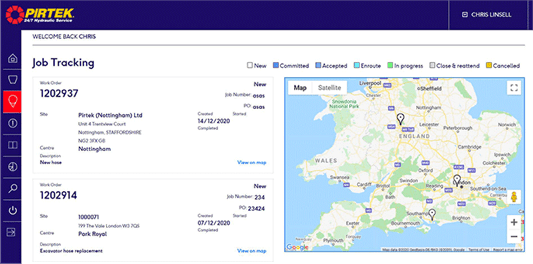The image is a screenshot of a web page set against a dark blue background. In the upper left corner, the company name "PeerTech" is prominently displayed in yellow text, alongside a donut-shaped red logo. The central part of the web page features a white rectangular area.

At the top left of this area, there is a greeting text that reads, "Welcome back, Chris." Below the greeting, "Job tracking" is displayed, indicating the purpose of the web page.

On the right side of the white rectangular area, there is a blurred map, which seems to depict a geographical region. Although the map is indistinct, it's apparent that it focuses on Wales, a country in the United Kingdom. Several locations in England are also visible, including Liverpool, Sheffield, and Plymouth. Additionally, a national park is identifiable in the upper left corner of the map, although its name is not legible.

To the left of the map, there is text that reads "PeerTech Nottingham Ltd.", indicating the name and location of the company.